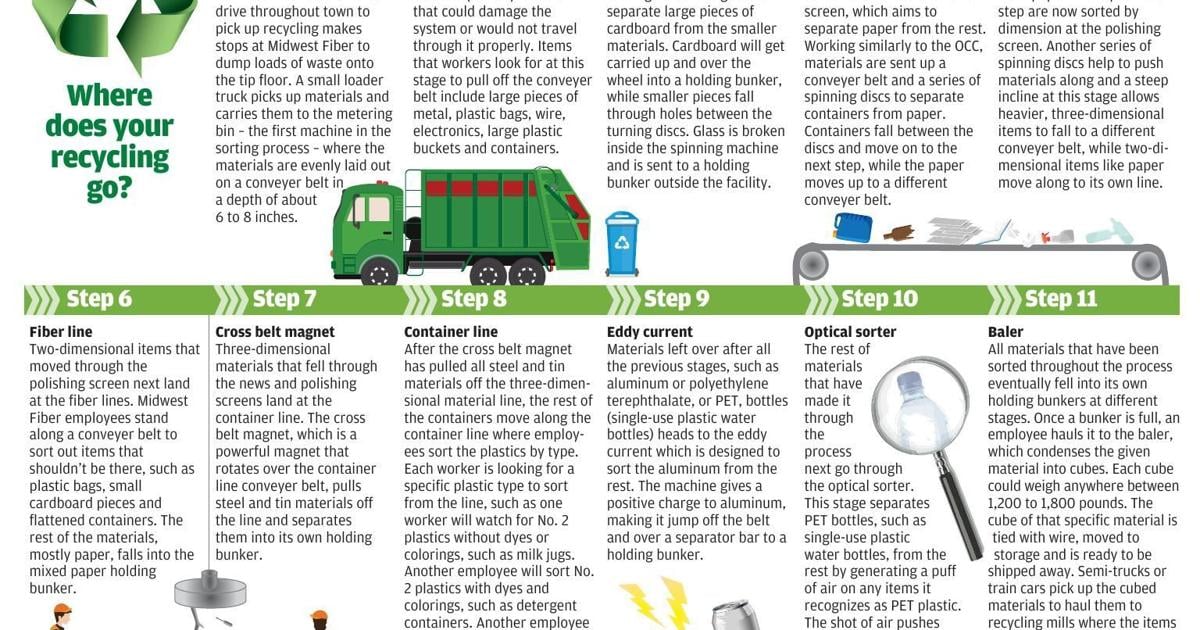This image is a heavily cropped screenshot of an infographic titled "Where Does Your Recycling Go?" occupying the top left-hand corner. It details steps 6 through 11 in the recycling process, illustrated within a vibrant green graphical framework. The steps are as follows: Step 6 - Fiber Line, Step 7 - Cross-Belt Magnet, Step 8 - Container Line, Step 9 - Eddy Current, Step 10 - Optical Sorter, and Step 11 - Baler. Each step is vividly associated with a specific graphic and a detailed text description, though much of the text is truncated due to cropping. Visual elements include a green garbage truck adorned with red stripes and black wheels, a blue recycling bin with a recycling logo, an assembly line or conveyor belt carrying recyclables such as broken glass pieces and empty bottles, and a magnifying glass examining a water bottle. The infographic uses concentric triangles to connect the steps, enhancing the visual flow from one to the next.